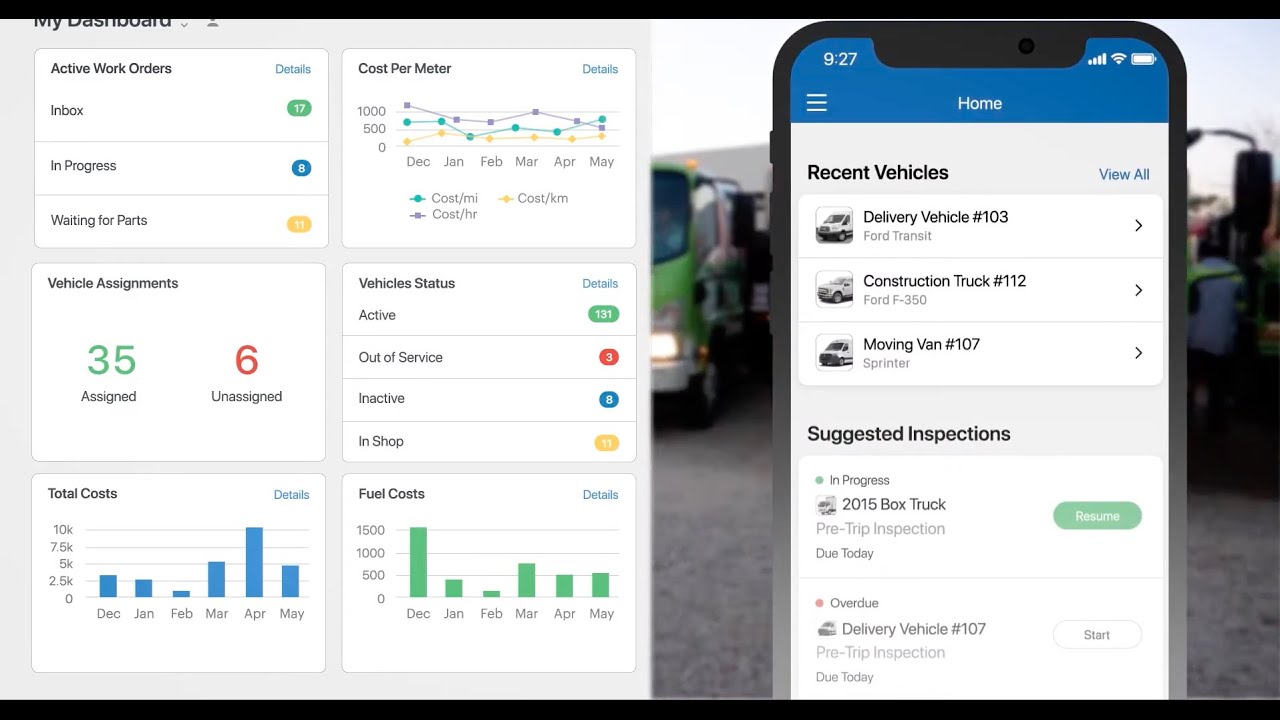The image features a screen capture of a detailed dashboard layout. On the left-hand side, the title "My Dashboard" is prominently displayed. Below, six white widget boxes are arranged in a two-column by three-row grid:

1. **Active Work Orders**: Summarizes the status with categories such as Inbox, In Progress, and Waiting for Parts.
2. **Cost Per Meter**: Shows a line graph depicting cost metrics (per mile, per hour, and per kilogram) from December to May.
3. **Vehicle Assignments**: Lists 35 vehicles as assigned and a further 6 in an assigned state.
4. **Vehicle Status**: Categorizes the fleet status into Active, Out of Service, Inactive, and In Shop, with corresponding numbers.
5. **Total Costs**: Presents a bar graph illustrating total costs over the months from December to May.
6. **Fuel Costs**: Another bar graph, depicting fuel costs during the same period.

On the right-hand side, a simulated mock phone screen displays a menu. This includes "Recent Vehicles" with three items listed below, and another section titled "Suggested Inspections" detailing two vehicles. In the background behind the phone screen, there’s a blurred-out image of trucks, adding contextual relevance to the dashboard's focus on vehicle management and cost tracking.